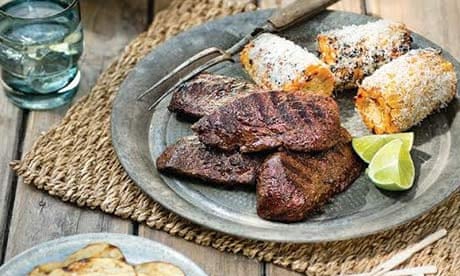In this color photograph, we see a rustic picnic setting with a brown wooden picnic table as the backdrop. Central to the composition is a woven brown wicker placemat, upon which a large gray plate is placed. The plate showcases a delicious spread of four thick pieces of grilled steak, complete with prominent grill marks. Accompanying the steaks are two lime wedges and three small pieces of grilled corn on the cob, dusted with a white, powdery seasoning that appears to be some kind of cheese, possibly elote. A two-pronged grilling tool is positioned beside the plate, indicating its use for handling the meat. In the upper left corner, set against the wooden planks, sits a blue transparent glass filled with clear water. Additionally, a fork with two tines rests on the table, and a partially visible metal plate with potato chips can be seen in the lower left corner, further enriching the picnic ambiance.